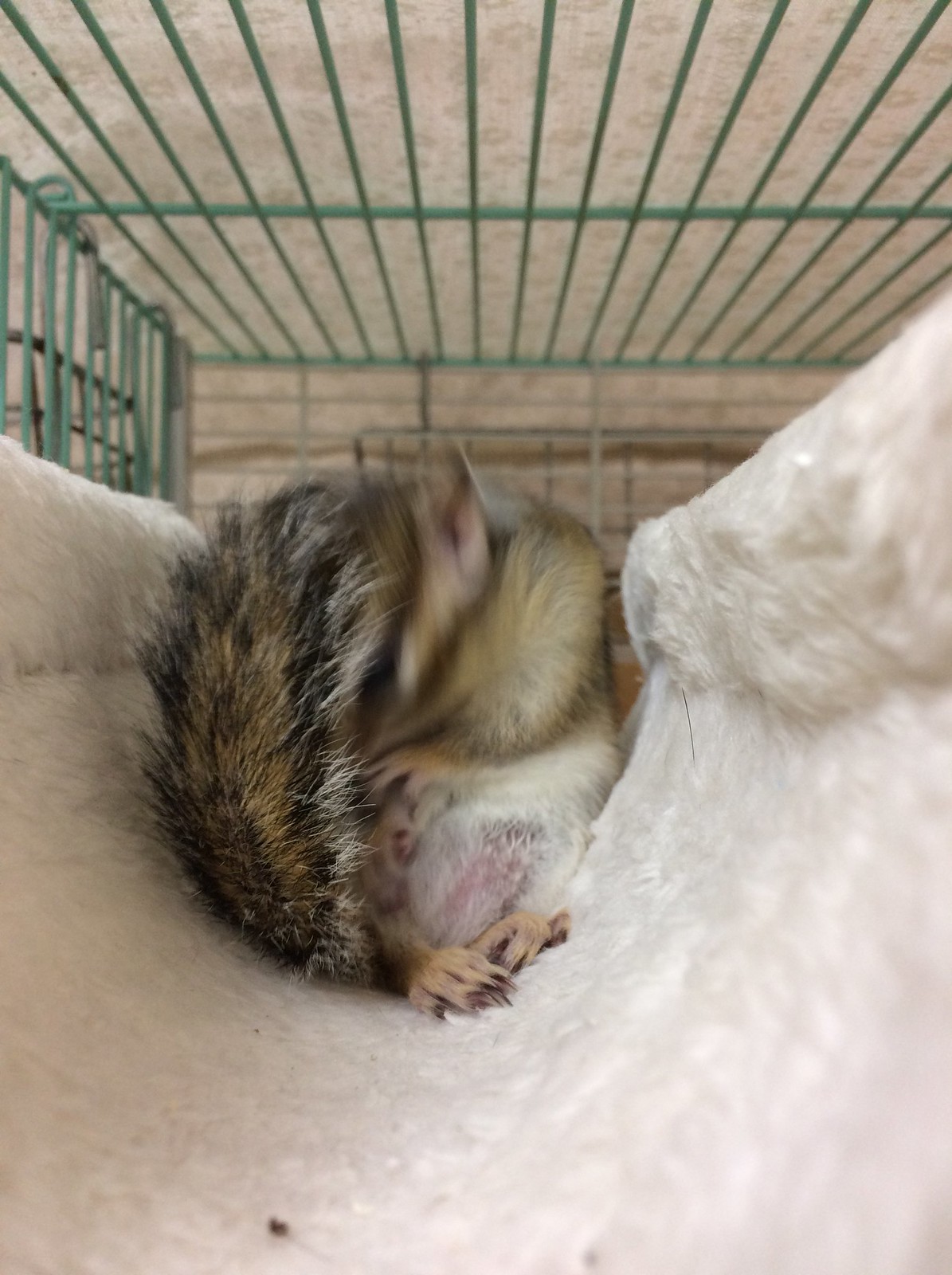This photograph captures a small rodent, likely a squirrel, nestled in a cozy white, fluffy bed. The animal, with a coat of brown, black, and white fur, is captured in motion, blurring its face as it tucks its head behind its tail. Its brown feet are faintly visible, peeking out from under its curled-up body. The fluffy bed, providing warmth and comfort, is situated inside a green cage, indicating that the rodent is a beloved pet. The overall scene evokes a sense of tranquility and care, highlighting the snug retreat of this charming creature.